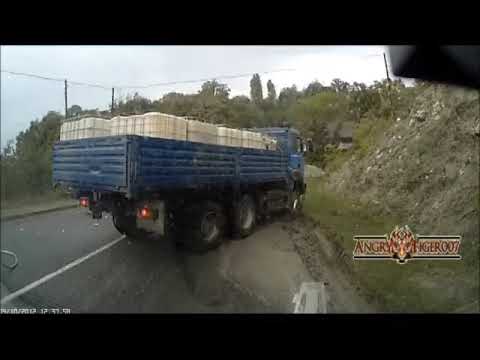The image depicts a blue flatbed truck with at least six wheels, carrying multiple large white water containers, veering towards the side of a paved, two-lane road. The road has a solid white line in the middle, bordered by grassy hills and dirt on both sides. The front tire of the truck appears to be stuck in the dirt as the vehicle is angled diagonally at approximately 45 degrees. Overhead, there are poles and wires, with trees and a partly cloudy sky visible in the background. The image has a black border on the top and bottom, and in the bottom right corner, there is reddish-brown text that reads "AngryTiger007" next to a symbol resembling a fiery face. The bottom left corner shows a date and time stamp: "14-10-2012 12-37-51".